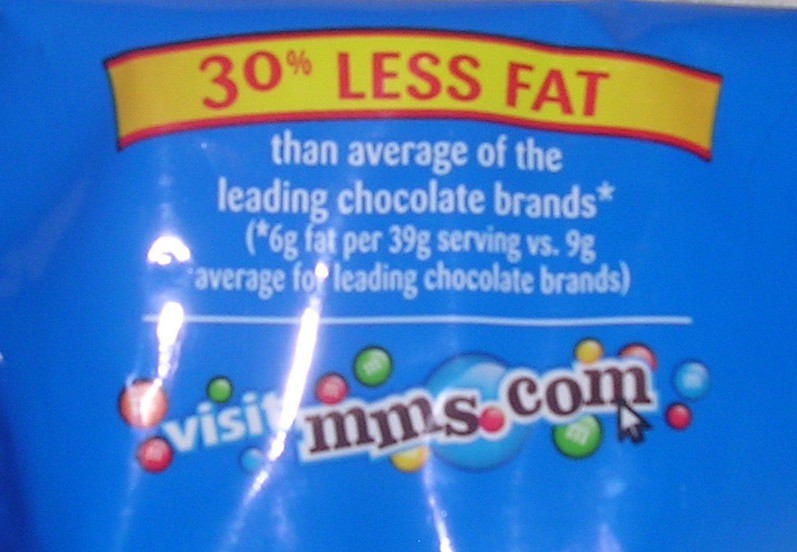This image captures a close-up view of a candy wrapper for M&M's, featuring a vibrant sky-blue background. Prominently displayed at the top is a yellow ribbon with red text that reads "30% less fat." Below this, in white font, it states, "than average of the leading chocolate brands," accompanied by a parenthetical note, "6 grams fat per 39 gram serving versus 9 grams average for leading chocolate brands." Further down, there's a white line separating this information from the text "visit mms.com." The lower part of the image showcases colorful illustrations of M&M's in green, orange, yellow, and red, each with the iconic "M" emblem. This detailed depiction highlights both the nutritional information and the vibrant design of the candy's packaging.